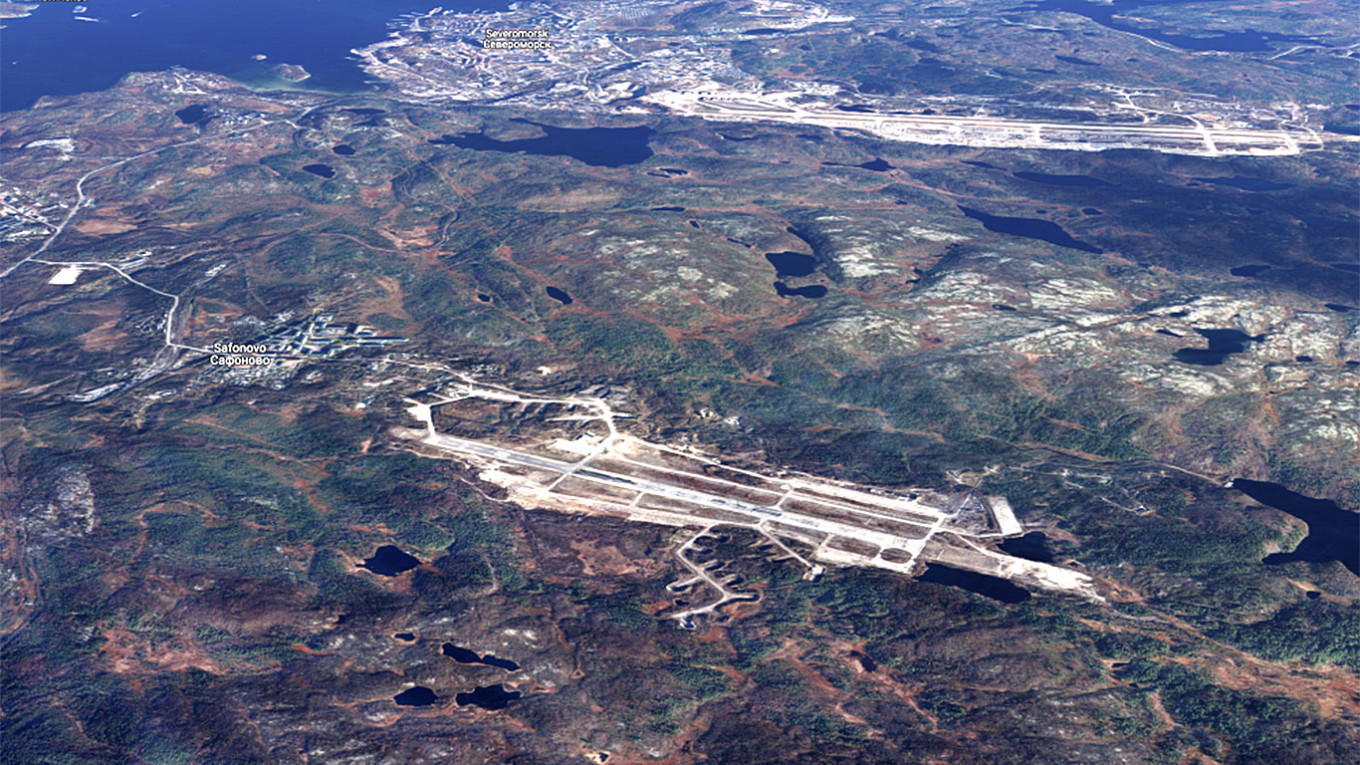The image is a high aerial photograph that captures a vast landmass predominantly featuring uninhabited terrain, with hues ranging from brown to green, likely representing varying vegetation types such as trees or brush. Scattered across the landscape are small bodies of water, with a notably larger water body in the upper left-hand corner that extends off the image.

In the upper section of the photograph, there are more man-made structures, possibly indicating a town or city, though the labeling is too tiny to decipher clearly. A prominent feature in the upper middle of the image is a structure that could be a highway or runway, stretching horizontally from left to right. Beside it, there are some hills and rocky formations. Another area potentially identifying as an airport or landing strip is visible towards the center, characterized by its white lines and concrete surface, though no buildings are immediately adjacent to it. Text within this area suggests the name "Salerno" or "SAFONOVO," but it is not entirely legible due to blending with the background.

In the middle left portion, there are more buildings, identified by small white text, yet they remain unreadable. The right side of the image exhibits darker green regions and additional small patches of water. The photograph overall showcases a mix of natural and human-made elements, providing a detailed view of the diverse landscape below.